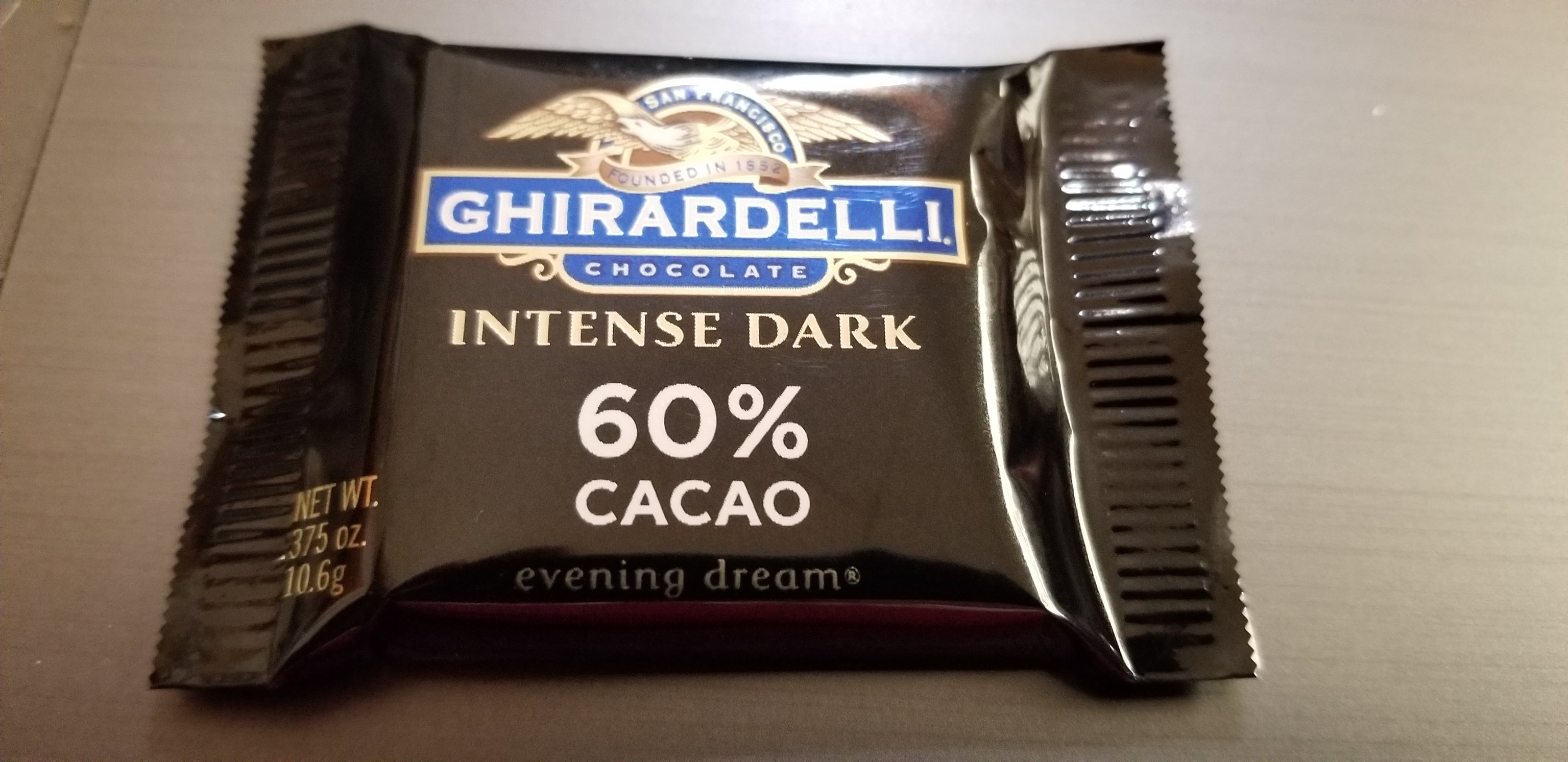The image showcases a close-up of a small packet of sweet, specifically a chocolate from the Ghirardelli brand. The packet is made of plastic and features a rich dark brown color with an orange hue. A subtle pinkish outline can be seen near the bottom of the packet.

The packet is slim and about the size of a small squash. At the top of the packet is the Ghirardelli insignia, followed by the brand name "Ghirardelli" in large text. Below the brand name, the words "Chocolate" and "Intense Dark" are printed, indicating the type of chocolate. Furthermore, the packet specifies that the chocolate contains "60% Cacao," with "Evening Dream" inscribed beneath it, likely referring to the flavor or variety.

On the left side of the packet, the net weight is displayed as "Net Wt. 0.375 oz (10.6 g)," providing detailed information about the quantity of the chocolate.